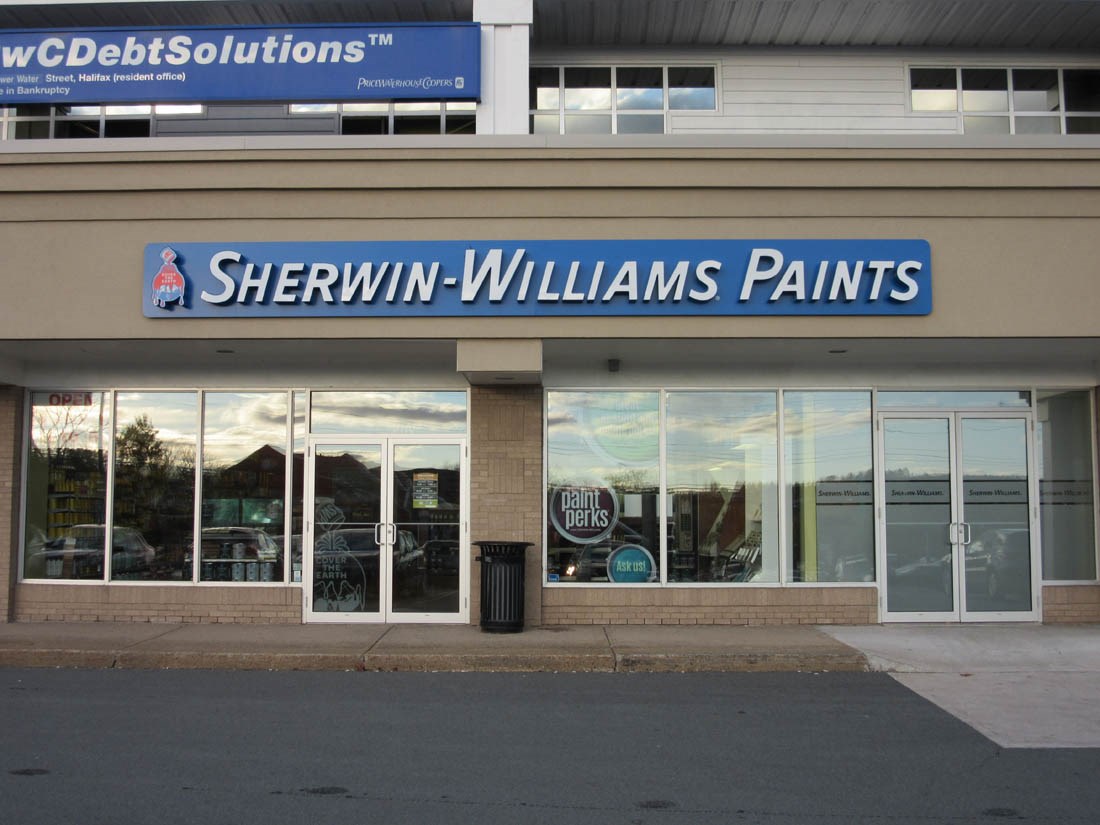The image showcases the upper section of a building where a walkway might be present. The building features white facades and very dark windows. On the left-hand side, there's a blue sign with white text that reads "WC Debt Solutions". Below that, another sign reads "Water Street Halifax Resident Office" with additional information about bankruptcy services. On the right-hand side, in a more elegant font, the words "Prince Water House Coopers" are displayed.

Further down, there is a Sherwin Williams sign depicting a blue globe being painted red with the slogan "Cover the Earth" in white. Towards the left, a set of double doors with very dark windows is visible. The building itself is constructed with light tan brick and darker gray concrete. To the right, another double set of doors, outlined in gray or silver, indicates a separate store, discernible by a white interior wall. The newer concrete in front of the exit is notably whiter and gray compared to the older concrete. Below this, the ground is covered with black asphalt, which has slick, dark spots that appear to be oil stains, adding an interesting texture to the scene.